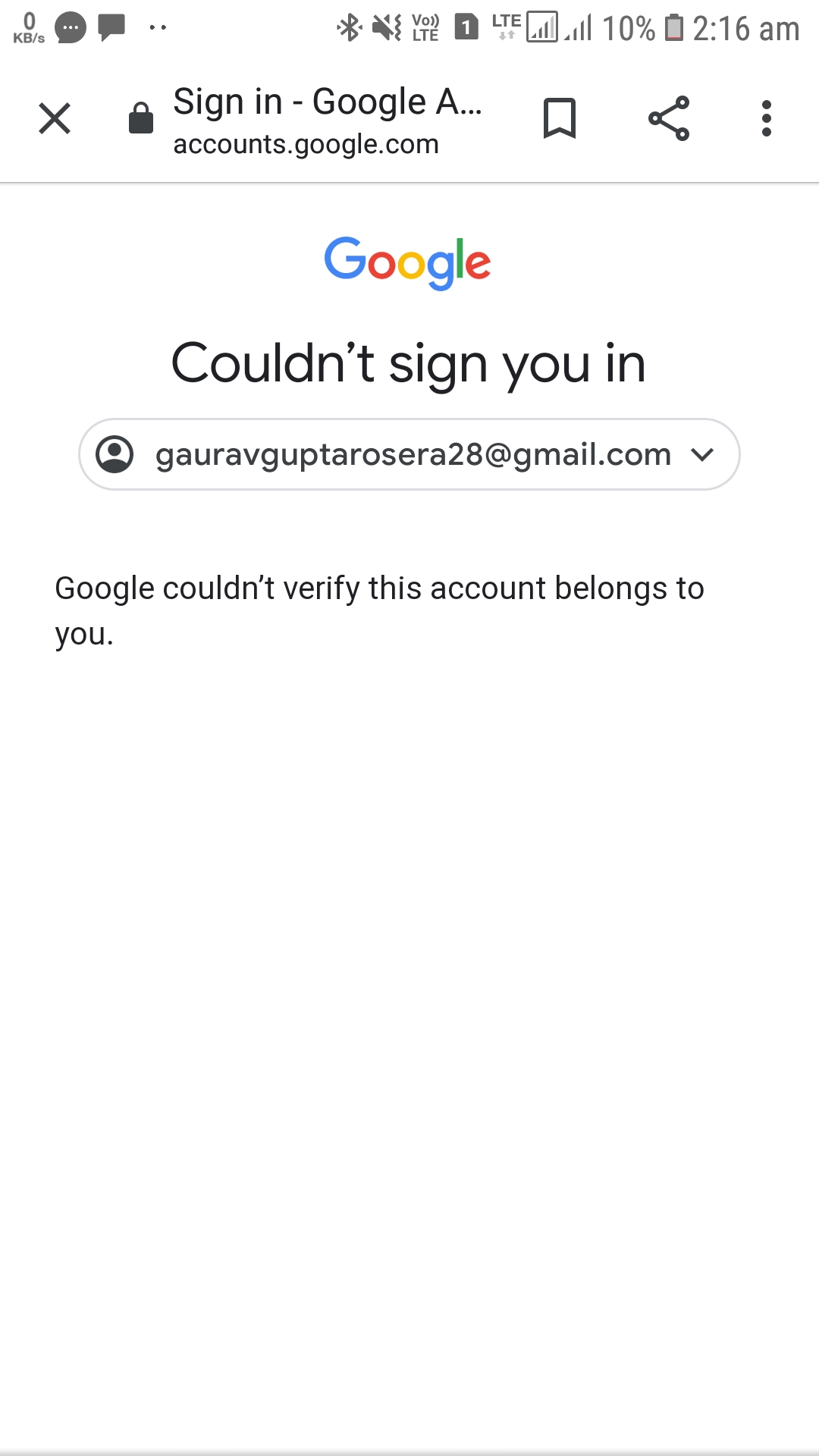**Screenshot Description: Google Sign-In Page**

- **Device Status Bar:**
  - **Left Side:**
    - Various phone icons including "0KB/s" and messaging icons.
  - **Right Side:** 
    - Bluetooth symbol
    - Silence icon
    - Partially visible box icon with the number '1'
    - LTE signal indicator
    - Signal strength bars
    - Battery icon displaying 10% charge
    - Time shown as 2:16 AM

- **Sign-In Page Content:**
  - **Top Section:**
    - A small 'X' icon
    - A lock icon
    - Bold text stating "Sign in - Google Accounts"
    - Web address shown as "accounts.google.com"
    - Icons for bookmarking, sharing, and additional options (three dots)
    - A faint gray separator line

  - **Main Content:**
    - Google logo with its iconic multi-colored letters (blue G, red O, yellow O, blue G, green L, red E)
    - Bold, black text indicating "Couldn't sign you in"
    - Drop-down menu with a user icon, displaying the email "gauravguptarose28@gmail.com"
    - A notification that reads: "Google couldn't verify this account belongs to you."